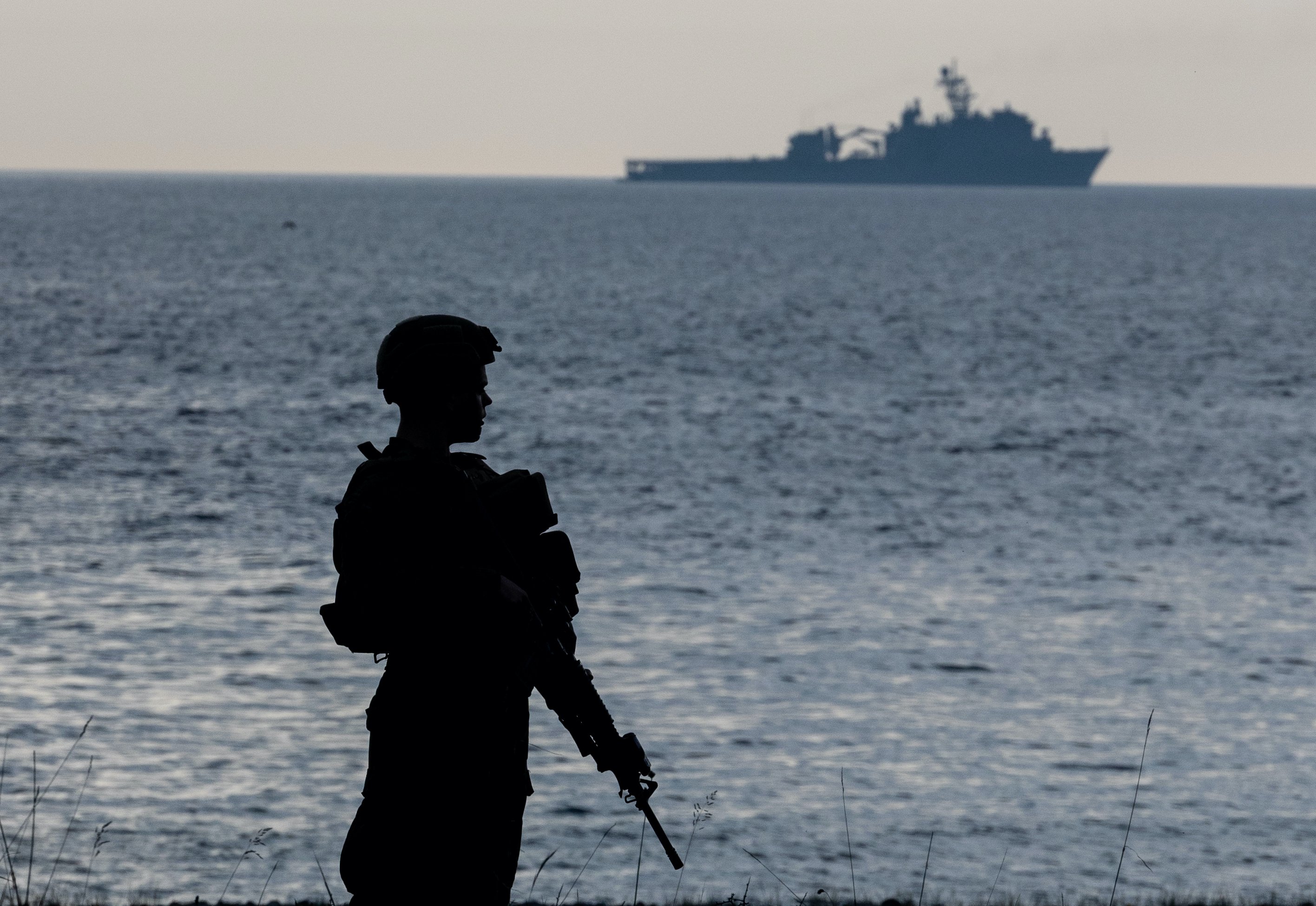This photograph captures a striking scene at dusk, showcasing a vast, choppy, bluish-gray ocean with the silhouette of a large naval warship on the horizon. The sky above, occupying the top fifth of the frame, is a brownish-gray, offering a stark contrast to the water below. The warship, slightly blurred and with a bluish tinge, appears massive and formidable, cutting through the light gray sky with a distinct, long, flat shape punctuated by noticeable humps.

In the foreground, dominating the left-center of the image, stands the silhouette of a soldier. The soldier's knees are cut off by the bottom of the frame, emphasizing their upper body. They are wearing a thick uniform with heavy body armor and a rounded helmet outfitted with goggles. Their stance is purposeful, slightly leaning back, possibly to balance the weight of the equipment strapped to their chest. The soldier holds a rifle, pointed downward at a slight angle to the right. This weapon is detailed, with the barrel just visible above the bottom edge of the image.

The bottom of the frame is lined with thin strands of grass, adding a natural touch to the otherwise stark and militaristic scene. Despite being in shadow, the soldier's profile is discernible, hinting at a young individual, possibly in their late teens or early twenties. Overall, the photograph combines elements of nature, human presence, and military might, all rendered in a cohesive, somber tone.